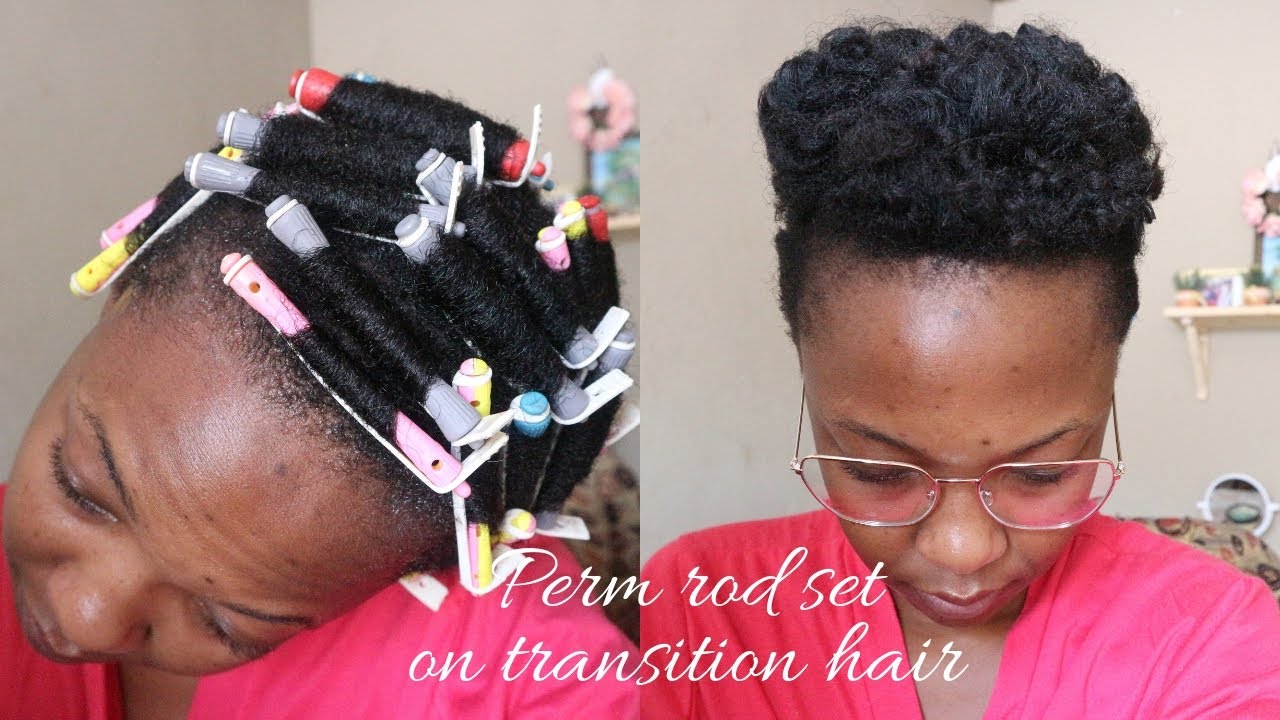The image consists of two color photographs of an African-American woman undergoing a hair transformation. In the left photo, she is wearing a pink top and tilting her head downwards to the right, showcasing an array of small, colorful curlers (pink, gray, white, and blue) secured with clips across her head. She is not wearing glasses in this picture. The backdrop appears to be a beauty salon with a beige wall. In the right photo, the same woman is seen with the curlers removed, revealing a beautifully styled head of curls atop her head. Now wearing glasses, she tilts her head slightly forward, emphasizing the curls. The bottom of the image features white text that reads, "Perm Rod Set On Transition Hair," suggesting a hairstyling process or tutorial.